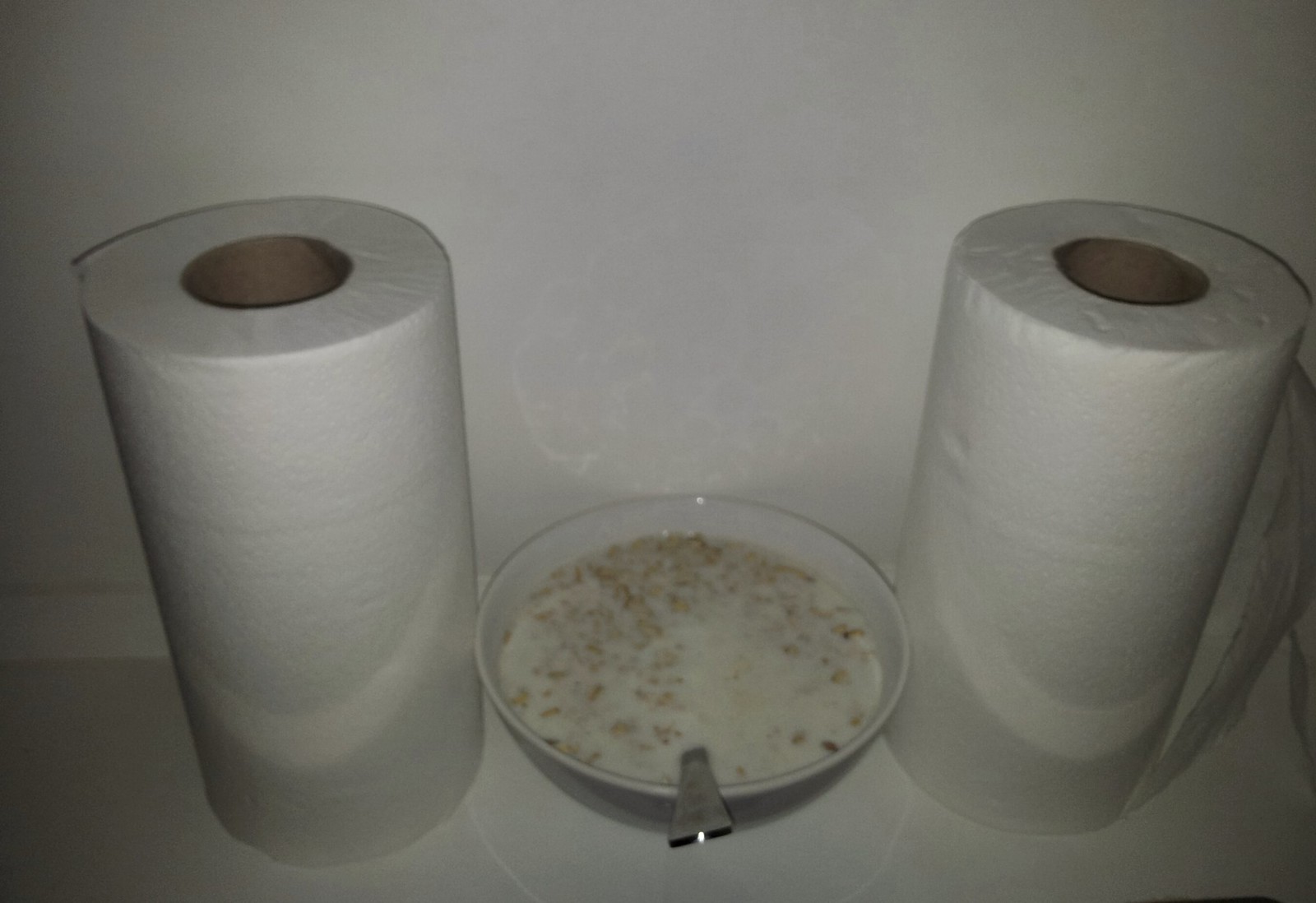The photo depicts a sparse and somewhat peculiar scene dominated by white hues. Central in the image, set against a white wall and on a white counter, is a white bowl brimming with milk. Submerged within the milk are visible brown specks of cereal, with a silver spoon protruding from the bowl. Flanking the bowl on either side are two new rolls of white paper towels, each featuring a conspicuous brown tube at the core. The shadows cast by the white elements give a slightly grayish tint, adding a subtle depth to the otherwise monochromatic composition. This real, unretouched photo, seemingly captured on a phone, evokes curiosity with its minimalism and utilitarian setup.